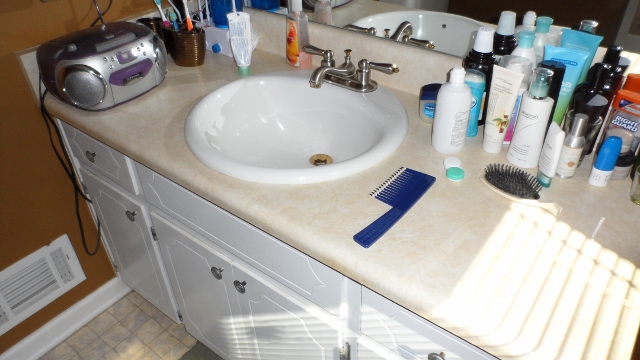In the image, a well-organized bathroom sink is captured, prominently featuring a marbled tile floor. The lower section of the sink showcases a spacious cabinet setup: two central bottom cabinets flanked by a door on either side, with two drawers on both the left and right sides separated by a middle section. 

In the bottom left corner of the image, a vent graces the tiled floor, presumably for heating or cooling. Atop the sink in the upper left-hand corner is a compact boom box, distinguished by its purple tape deck and rounded speakers, with a silver front and dark grey back. 

Nearby, there are three brass cups holding a trio of toothbrushes: one white and blue, one blue and baby blue, and one orange and white. Adjacent to these, on the far right, sits a bottle of toothpaste and a bottle of hand soap. The sink itself is a bowl design equipped with a silver faucet that has distinct hot and cold handles, and a large mirror is mounted above it, reflecting the entire arrangement.

To the right of the sink, a blue comb and a white brush are placed alongside a pair of contact lens storage pods. A variety of skincare and hygiene products are organized in this area, including cough syrup, skin exfoliators, Right Guard deodorant, Speed Stick, and a container of petroleum jelly or possibly Vicks VapoRub situated at the back.